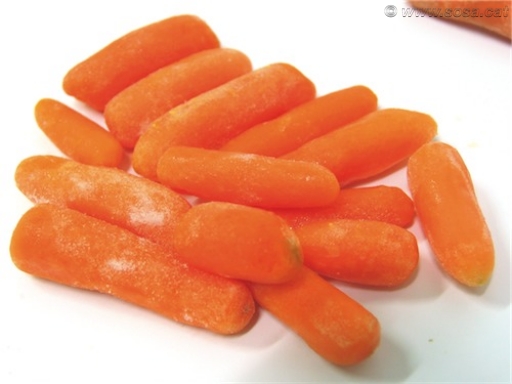This close-up color photograph features a collection of approximately 14 to 15 baby carrots arranged haphazardly on what appears to be a white cutting board or kitchen surface. The perspective is slightly wider than tall, showing the carrots positioned at various angles. A distinctive row of five carrots stretches diagonally from the top left corner towards the bottom right, oriented around 2 o'clock. Adjacent to the far-right carrot in this row is one carrot forming the top of a triangle, pointing approximately at 11:30. The remaining carrots are laid out horizontally, with most appearing sporadically stacked on one another, and some notably small ones dispersed throughout. Only two carrots possess green marks where stems had been, one positioned near the right side of the horizontal grouping and another near the triangle's base. The image's overall color appears slightly washed out, likely due to overexposure, with some visible shimmer indicating potential flash usage. The surface’s faint writing hints at a brand or manufacturer name, adding a subtle contextual layer to the scene.